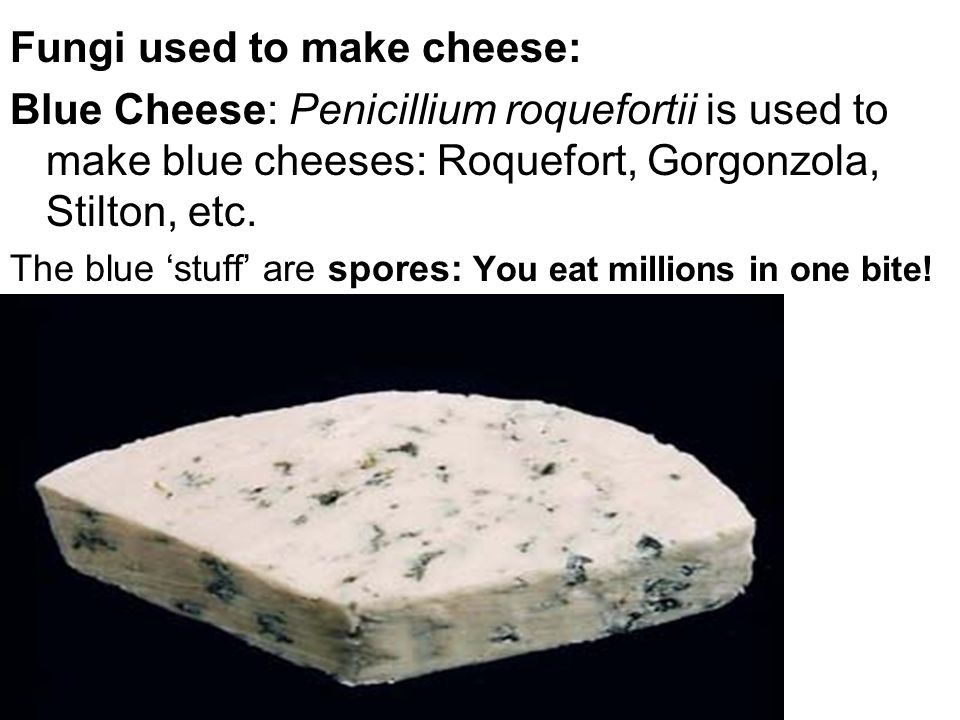The image features a detailed composition consisting of two primary elements: a caption and a photograph. The black and white caption at the top reads: "Fungi used to make cheese. Blue cheese. Penicillium roqueforti is used to make blue cheeses such as Roquefort, Gorgonzola, Stilton, etc. The blue stuff are spores— you eat millions in one bite!" The text is predominantly black on a white background, with portions of it bolded and italicized for emphasis.

Below the caption, the photograph captures a slice of blue cheese set against a stark black background. The cheese appears as a wedge, resembling a slice of bread with three square sides and a rounded top. The white body of the cheese is intricately marbled with greenish-blue veins and chunks, which are clarified in the caption as spores of Penicillium roqueforti.